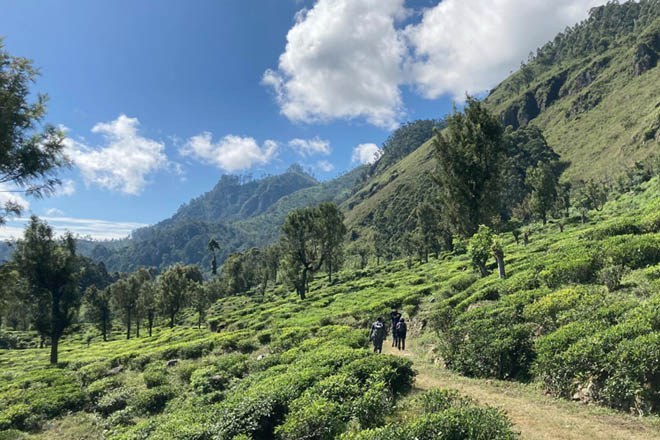The image depicts a picturesque and rugged hiking trail known as the Pico Trail in Sri Lanka, renowned for its tea plantations. The trail winds through a steep hillside adorned with lush greenery, including rows of short green shrubs and dispersed full-grown trees with dark green leaves. The dirt path is well-trodden and free of tall vegetation, guiding a group of hikers, some wearing blue with visible white logos. Further back, a small mountain range rises majestically, its lower slopes blanketed by dense foliage. The background showcases a stunning vista of a light blue sky dotted with two large white clouds and several wisps of smaller clouds. Branches with dark green leaves peek into the top left corner of the image, adding to the sense of immersion in this remote, vibrant natural setting.